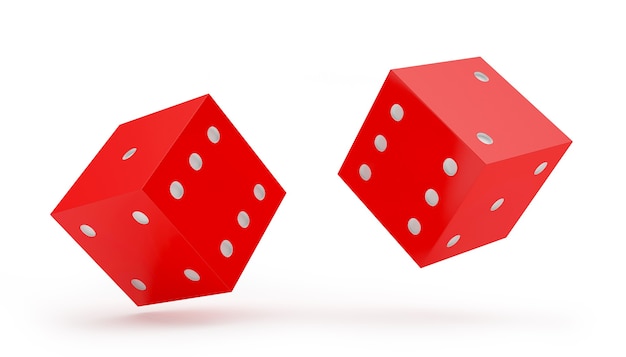In this detailed image, we see a pair of red dice with white pips, seemingly suspended in mid-air against a white background. Both dice appear to be floating, casting small shadows beneath them, which suggests they've just been thrown and are descending towards the surface. The dice are depicted with a high degree of realism, possibly in a computer rendering. 

On the left die, the number six faces the right side with a one on top and a four at the bottom. Conversely, the right die also shows a six, but with a two on top and a three to the side. The transparency and detailed texture of the dice give them a nearly ethereal appearance, emphasizing their red color and the contrasting white pips. The orientation of the dice suggests that their positions may change as they land, adding a sense of anticipation to the scene.